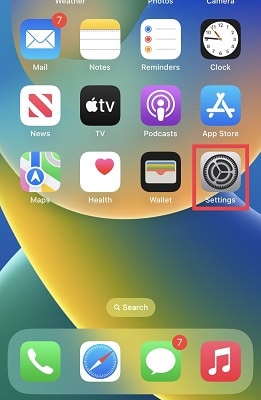This image is a cropped screenshot taken from a cell phone, with the top portion slightly cut off. The phone's background wallpaper features a vibrant swirl of blue, orange, and yellow colors. Moving from the top of the screenshot downward:

1. The **Mail** application is depicted as a blue square with a white envelope icon in the center. A red circle in the top right corner of the square indicates there are seven unread messages.
2. The **Notes** application has a yellow banner at the top of the square followed by two thin, gray horizontal lines beneath it.
3. The **Reminders** application displays as a bullet point list with blue, red, and yellow bullet points.
4. The **Clock** application icon features a clock face.
5. The **News** application is a square made up of diagonal red and white stripes.
6. The **TV** app icon is a black square showcasing the Apple logo—a white apple with a bite taken out of the left side—and the word "tv" in lowercase letters.
7. The **Podcasts** application is represented by a white microphone icon surrounded by two circles.
8. The **App Store** icon displays a white "A" on a blue square background.
9. The **Maps** app presents a miniature map illustration.
10. The **Health** app shows a white square with a red heart in the top right corner.
11. The **Wallet** app icon is a black square featuring the image of a wallet.
12. The **Settings** app is depicted as a gray square with a black gear icon in the center, and this item is outlined in a red square.

At the bottom of the screenshot, there's a "Search" bar. Additionally, there are four key icons on a dock:
- **Phone**
- **Safari**
- **Messages**, with a count of seven unread messages indicated by a red badge.
- **Music**